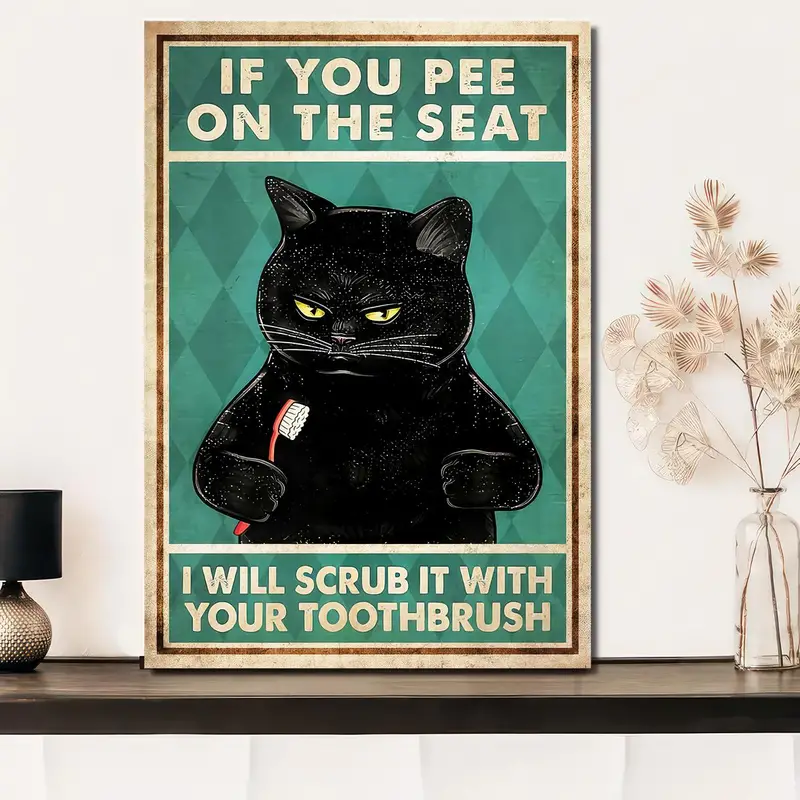The image shows a detailed, humorously captioned canvas propped against a stark white wall, resting on a sleek black shelf. The canvas, outlined in tan, sports an engaging harlequin check background with alternating tones of green and dark green. Boldly inscribed in beige at the top of the canvas are the words, "If you pee on the seat," and at the bottom, it forewarns, "I will scrub it with your toothbrush." Central to the artwork is a whimsical drawing of a pudgy black cat with yellow eyes, wielding a red toothbrush in its right woodpaw, giving off an air of stern admonition. The scene is flanked by a short table lamp on the left and a tall clear vase with dried grass on the right, creating a balanced, aesthetically pleasing display.